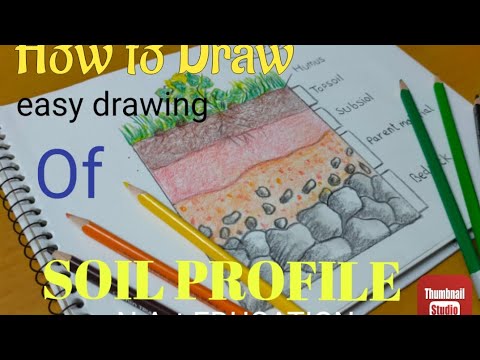The image is a thumbnail for a YouTube video titled "How to Draw Easy Drawing of Soil Profile." The title spans large fonts with "how to draw" in yellow, "easy drawing" in black, "of" in purple, and "soil profile" in yellow. The background features black rectangles at the top and bottom. A sketchpad, partially cut off at the top and bottom, is angled diagonally and shows a detailed diagram of soil layers ranging from grass to dirt, reddish dirt, orange dirt with small gray rocks, to bedrock at the bottom. The layers, labeled as humus, topsoil, subsoil, and bedrock, are illustrated with colored pencils placed on the sketchpad: brown, orange, and yellow on the left, and two shades of green and black on the right. In the lower right corner, there is a partially visible logo resembling the YouTube logo, labeled "Thumbnail Studio."